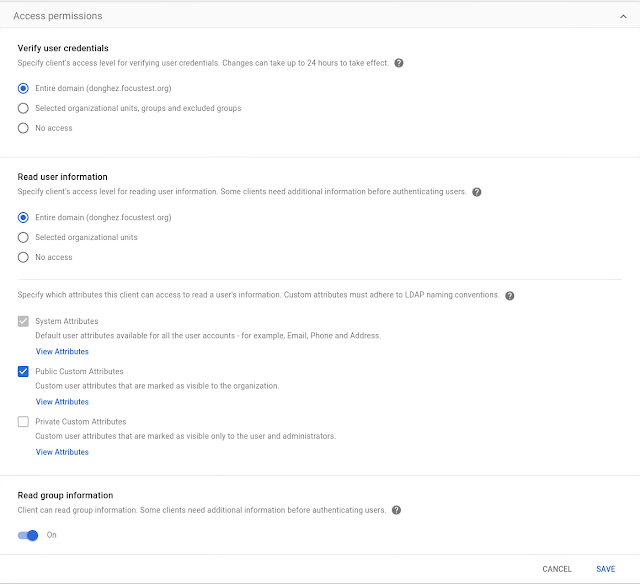The image depicts a webpage displayed on a tablet, likely an iPad. Dominating the top of the page is a header that reads "Access Permissions," accompanied by a directional arrow. The main content is elegantly laid out on a white background with crisp black lettering. To the left are several selectable blue buttons, each representing a different access permission option. These permissions include: verifying user credentials, reading user information, specifying attributes, and reading group information. Adjacent to each permission is an on/off toggle switch for enabling or disabling the respective settings. Additionally, small question mark icons are present, offering users helpful instructions and explanations about each permission. At the bottom of the page, two prominent buttons labeled "Cancel" and "Save" allow users to either discard changes or save their configured settings.